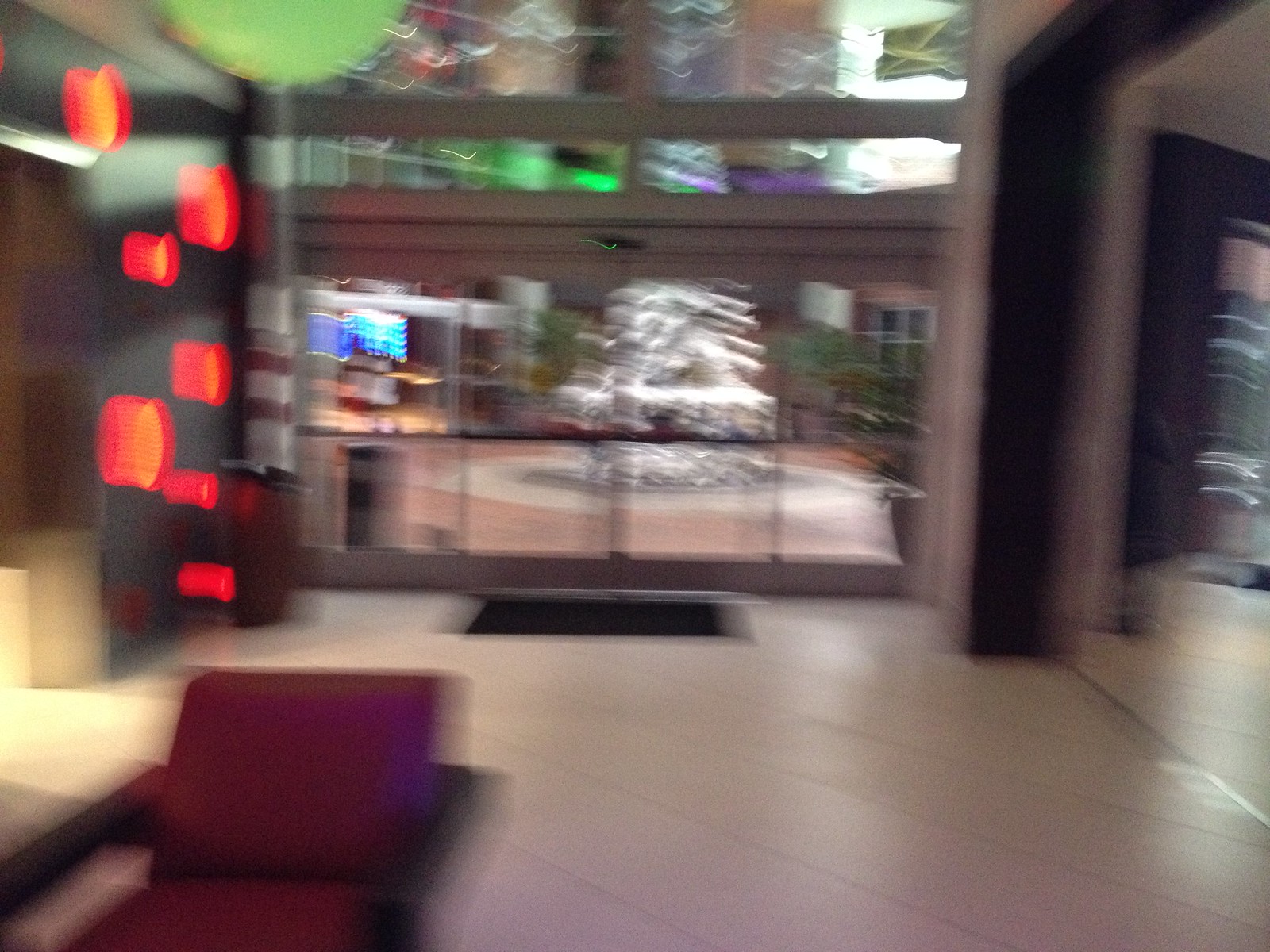The image appears to depict the lobby of a shopping plaza, captured with a pronounced blur. On the left side, there is a structure that resembles an elevator set against a dark brown wall. The wall features large, round, red circles which might be elevator buttons or decorative elements, though they are indistinct due to the blurriness. The floor is made of beige tiles, with a brown mat positioned centrally. In the middle of the image are large glass doors, through which a prominent white flocked Christmas tree is visible, indicating holiday decor. Beyond these glass doors, various stores and lights can be discerned, further suggesting that this is a bustling retail area. An additional entrance can be seen to the right, reinforcing the setting of a shopping plaza lobby.